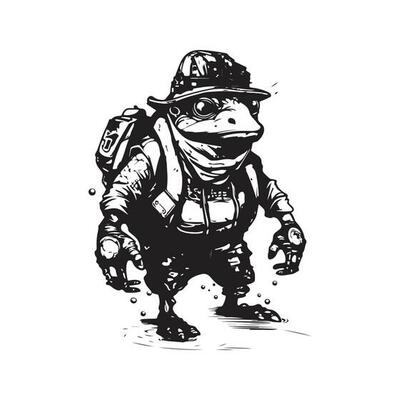This is a highly detailed black and white pencil drawing of an anthropomorphized toad standing upright on its hind legs. The toad is dressed in a combination of miner, cave explorer, and steampunk-style attire. On its head, it dons an old-fashioned fireman's hat, adorned with a bouquet of steampunk-inspired flowers on the front bill. The toad's face features typical toad characteristics, such as large eyes and a beak-style muzzle, with its mouth open as if talking or catching raindrops. 

The amphibian is clothed in a long-sleeved shirt and pants, with distinctive steampunk gloves on its hands, which hang down by its sides. It wears a square backpack on its back. The toad is barefoot, standing amidst some black streaks and water droplets, suggesting a rainy environment or perhaps that it has recently emerged from water. The toad's overall appearance and attire hint at a role as a miner or cave explorer, navigating challenging terrains and weather conditions.